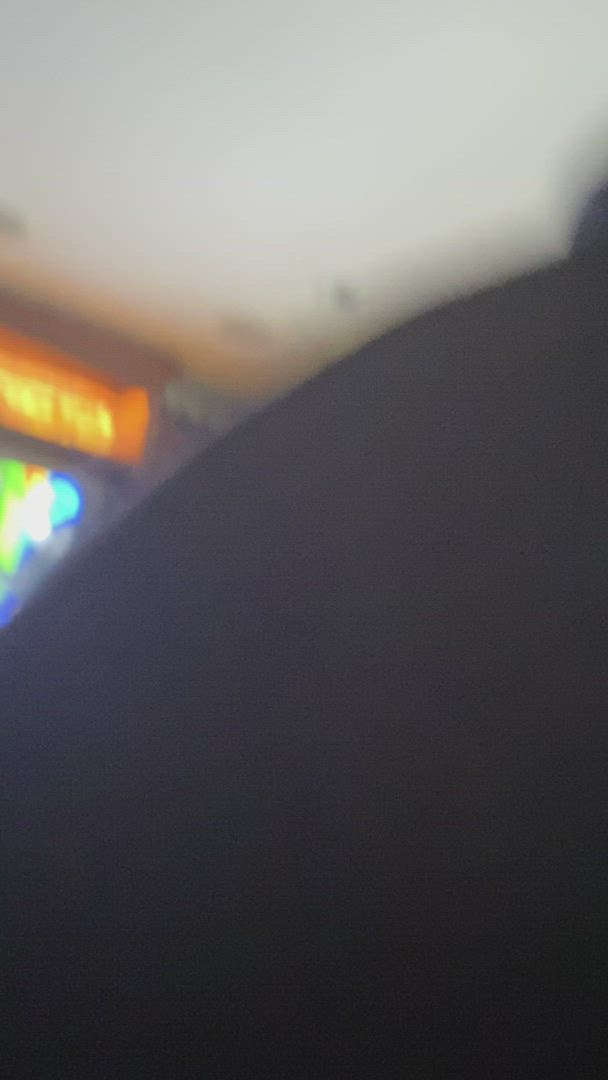This photograph appears to have been taken by accident or during someone's movement, resulting in a heavily obscured image. The majority of the photo, approximately 70%, is dominated by a dark area that sweeps from the middle of the left side to nearly the top right corner, possibly caused by a person's hand, back, or shoulder blocking the camera. The visible portion of the image is confined to the top left corner and reveals a blurry scene. Here, a rectangular lit section with an orange background and illegible yellow writing is visible, suggesting it might be a sign, potentially from a restaurant or shop. Below this, there is a multicolored lit area featuring bright shades of blue, green, orange, and white, reminiscent of neon lights or a stained glass-like display. The rest of the scene just glimpses a white ceiling, enhancing the indoor setting’s probability. Despite the blur and obstruction, the patchwork of lights hints at a vibrant environment, possibly a commercial area.